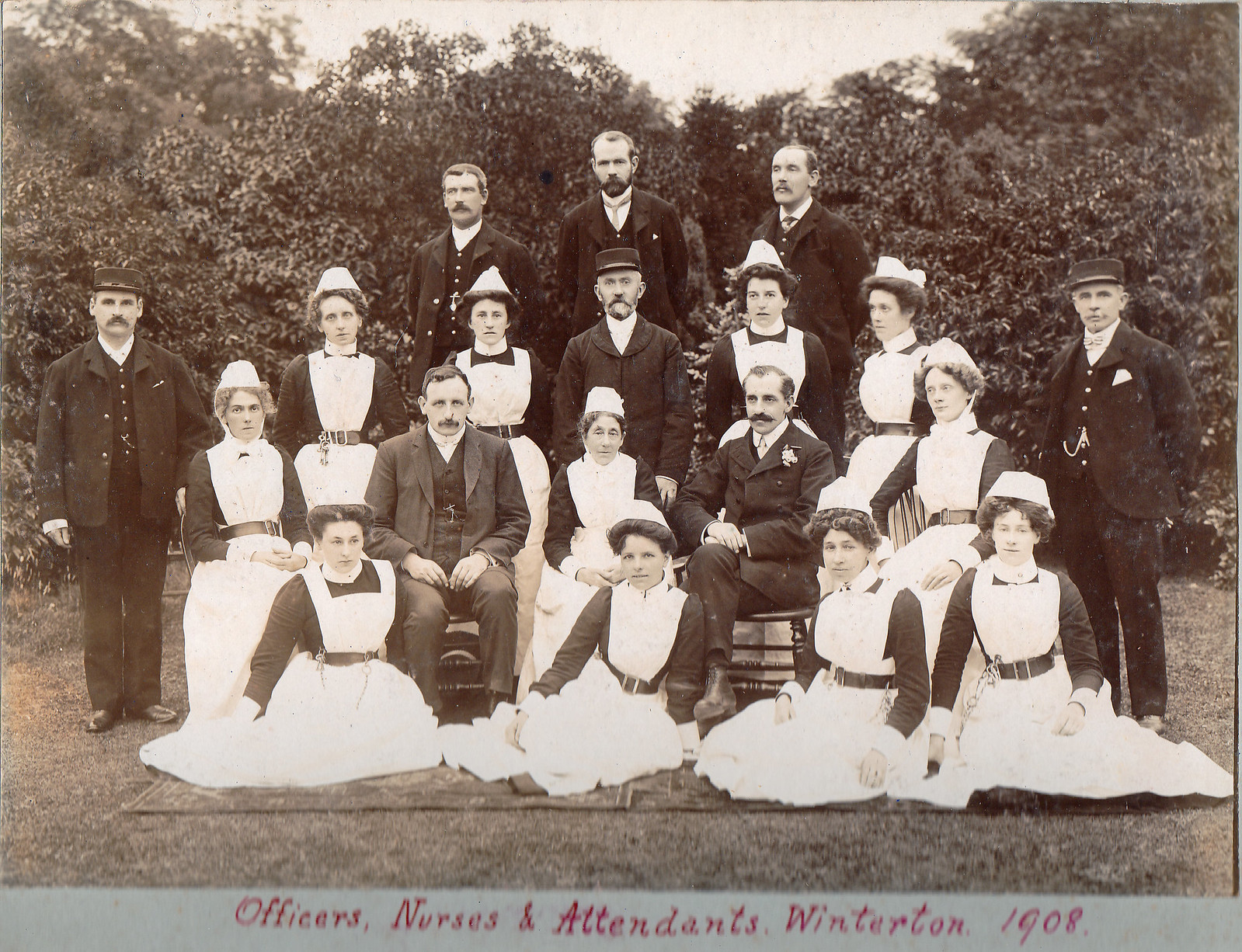This black-and-white photograph from 1908, captioned "Officers, Nurses, and Attendants, Winterton," features a large group of people arranged in distinct rows in an outdoor setting. In the front, four women, dressed in what appear to be white dresses and caps, are seated on the ground with their legs folded to the sides on a rug. Directly behind them, a row of people seated on chairs includes a mix of men and women. Specifically, starting from the left, there is a woman, a man, another woman, another man, and two more women, all the women in white uniforms and the men in suits. Flanking this row are two men standing on either end.

The next row up consists of individuals standing: three men and four women, continuing the attire pattern with the women in white uniforms and the men in suits. At the back, three more men, likely standing on elevated chairs or platforms to be visible, are also dressed in suits. Tall bushes form the background of the image, rising above the heads of the people and extending up to the top where bits of the sky can be seen. The bottom border of the photo features a blue background with the caption prominently displayed in red letters: "Officers, Nurses, and Attendants, Winterton 1908."